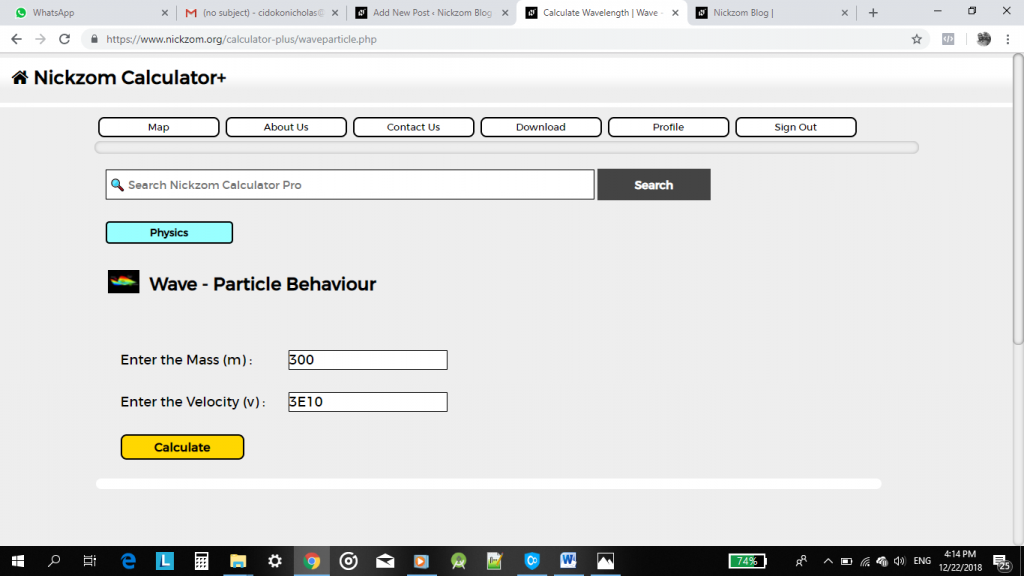Here is a detailed and cleaned-up descriptive caption for the image:

---

The image depicts the interface of an online calculator application named "Nik Zom Calculator Plus," displayed on a computer screen. The aspect ratio of the image is wider than it is tall. At the bottom of the screen, a black taskbar features application icons, notably Internet Explorer and Google Chrome, with Google Chrome currently active. There are approximately a dozen icons, and on the right-hand side, the system tray shows a battery percentage of 74% along with various status icons. The date and timestamp indicate it is 4:14 p.m. on December 22, 2018.

In the web address bar, "Nik Zom Calculator Plus" is prominently displayed, confirming the application's name. The browser has five open tabs, with the active one titled "Calculate Wavelengths Wave." Directly beneath the application's name, there are navigation buttons labeled "Map," "About Us," "Contact Us," "Download Profile," and "Sign Out." A search bar labeled "search Nik Zom Calculator Pro" is positioned to the right, accompanied by a blue search button.

The main content area features a blue rectangular header labeled "Physics" with a subtitle "Wave Particle Behavior." The interface prompts the user to "Enter the mass in meters," where the value "300" is entered in a text box. Following this, there is another prompt to "Enter the velocity, V," with "3E10" entered in the subsequent text box. The interface includes a yellow "Calculate" button, indicating that this portion of the calculator is designed to process some aspect of wave-particle physics.

---